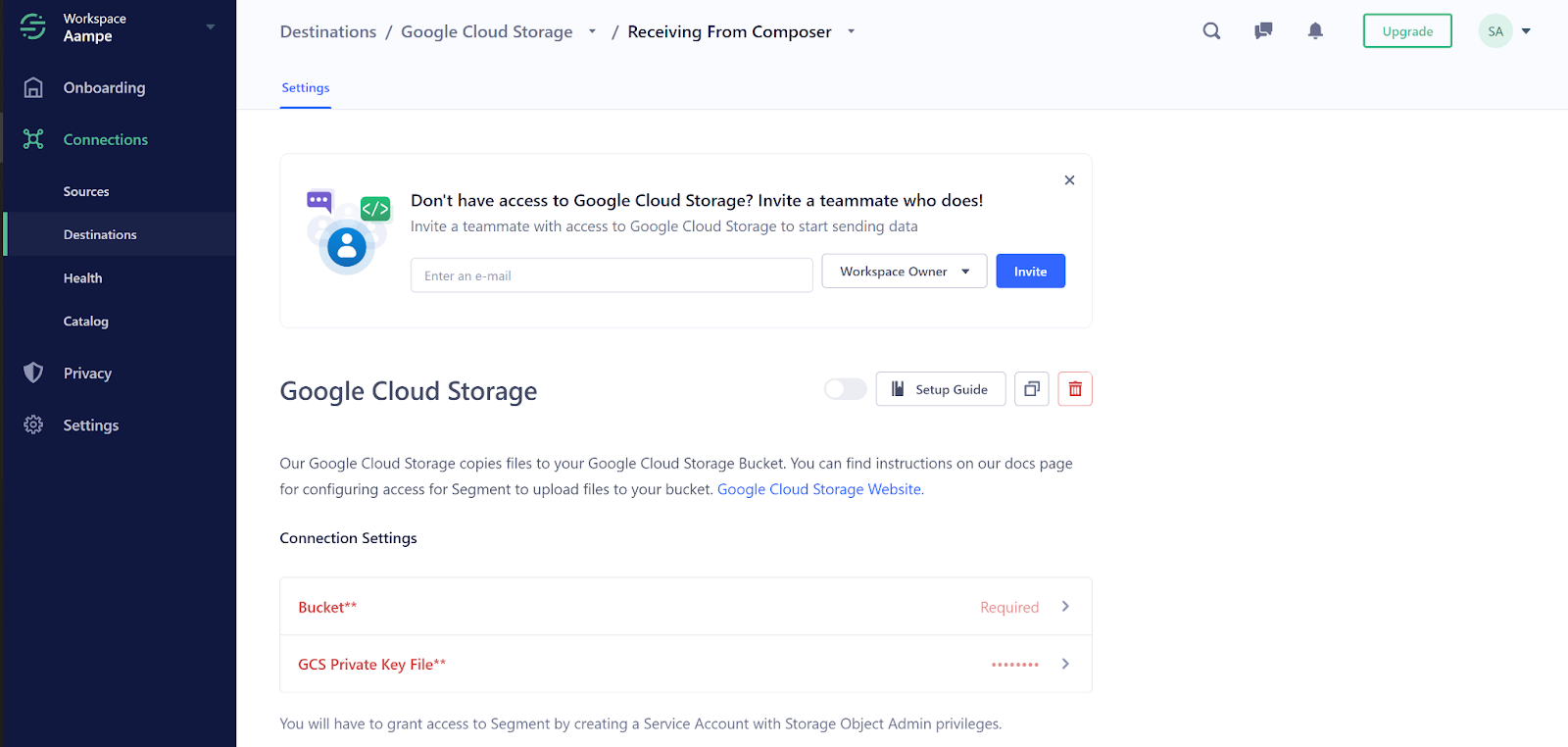The image displays a detailed interface for setting up Google Cloud Storage within a workplace environment, likely from a cloud services dashboard.

At the top of the screen, the word "Workplace" is prominently highlighted, alongside an "Amp" symbol, indicating the current workspace or environment. A navigation bar includes icons such as a magnifying glass for search, a speech bubble for messages, and a bell for notifications. There's also an "Upgrade" option visible.

Under the settings section, multiple text labels mention "Google Cloud Storage." One notification indicates the current user doesn't have access to Google Cloud Storage and suggests inviting a teammate who does. It advises you to email the workplace owner to gain access. A button labeled "Invite" is visible.

A "setup guide" for Google Cloud Storage is prominently displayed, explaining how to copy files to your Google Cloud Storage bucket. Instructions for configuring access and uploading files are available on their documentation page. Text on the website guides users through connection settings, highlighting a red-text term "bucket."

A section shows "GTS private key file," marked by an asterisk, explaining the necessity to grant access to a segment by creating a service account with storage object privileges. This area is part of the overall onboarding process, covering different tabs like Connections, Sources, Destination, Health, Catalog, Privacy, and Settings in various text styles and colors.